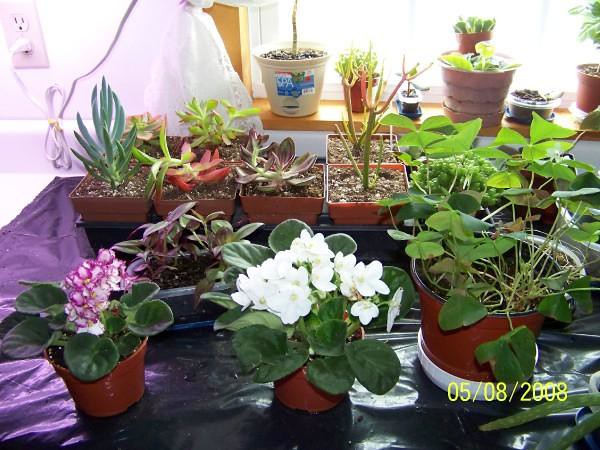The photograph, dated either May 8th, 2008, or August 5th, 2008, is an amateur shot capturing a brightly-lit work area filled with various potted plants. The center of the image features a table covered with black plastic, upon which an assortment of plants in different sizes and shapes of pots are displayed. Notably, there are several terracotta pots containing green leafy plants, some with white flowers and others with purple-tinged blooms. Alongside these, square pots and smaller black pots host a variety of succulents and other plant types.

In the background, more plants are positioned on a windowsill, bathed in sunlight streaming through an open window, highlighting the numerous potted cacti and ivy plants that close at night. An electric cord is seen plugged into a lower socket of an outlet, slightly off-frame to the side. The detailed assortment of plant life and the bright, natural light create a warm and busy horticultural scene, all dated clearly with "05/08/2008" in the bottom right of the image.